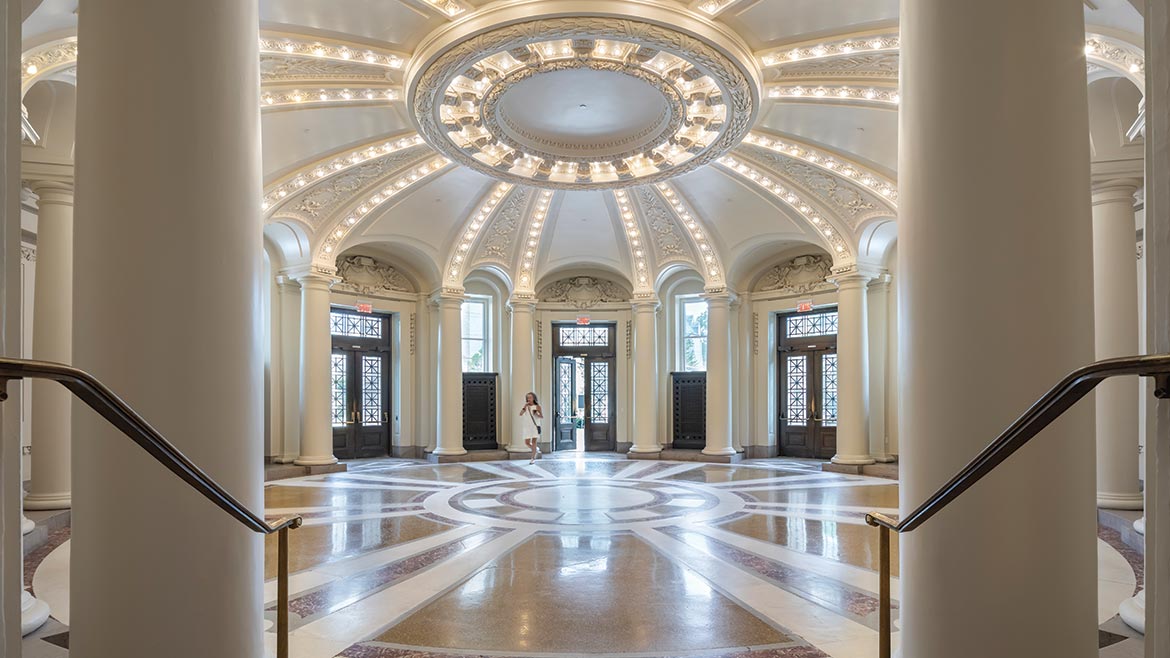The image captures the interior of an elegant, expansive, and ornately designed building, characterized by a harmonious blend of classic and modern architectural elements. The central feature of the space is its grand circular motif, which is prominently displayed both on the floor and the ceiling. The floor is primarily a light brown, shiny marble with a striking white circular pattern at its center, from which stylized rays extend outward, resembling rays of sunshine. Each ray is meticulously inlaid to create an intricate design that complements the overall circular theme.

White columns are strategically placed throughout the space, enhancing the grandeur and symmetry of the room. The ceiling mirrors the floor's circular design but with added ornate moldings and circular light fixtures that radiate outwards, creating a sophisticated, illuminated ambiance. Black railings flank the steps that lead into this majestic room, adding a contrasting element to the predominantly white interior.

At the far end of this large, round chamber, three evenly spaced, imposing black double doors stand, each framed by archways that echo the circular design motif. A young woman in a white dress is seen walking through the central double doors, her presence adding a touch of human connection to the grandeur of the space.

This setting evokes a modern interpretation of Victorian style, blending classic architectural elegance with contemporary lighting and design elements.